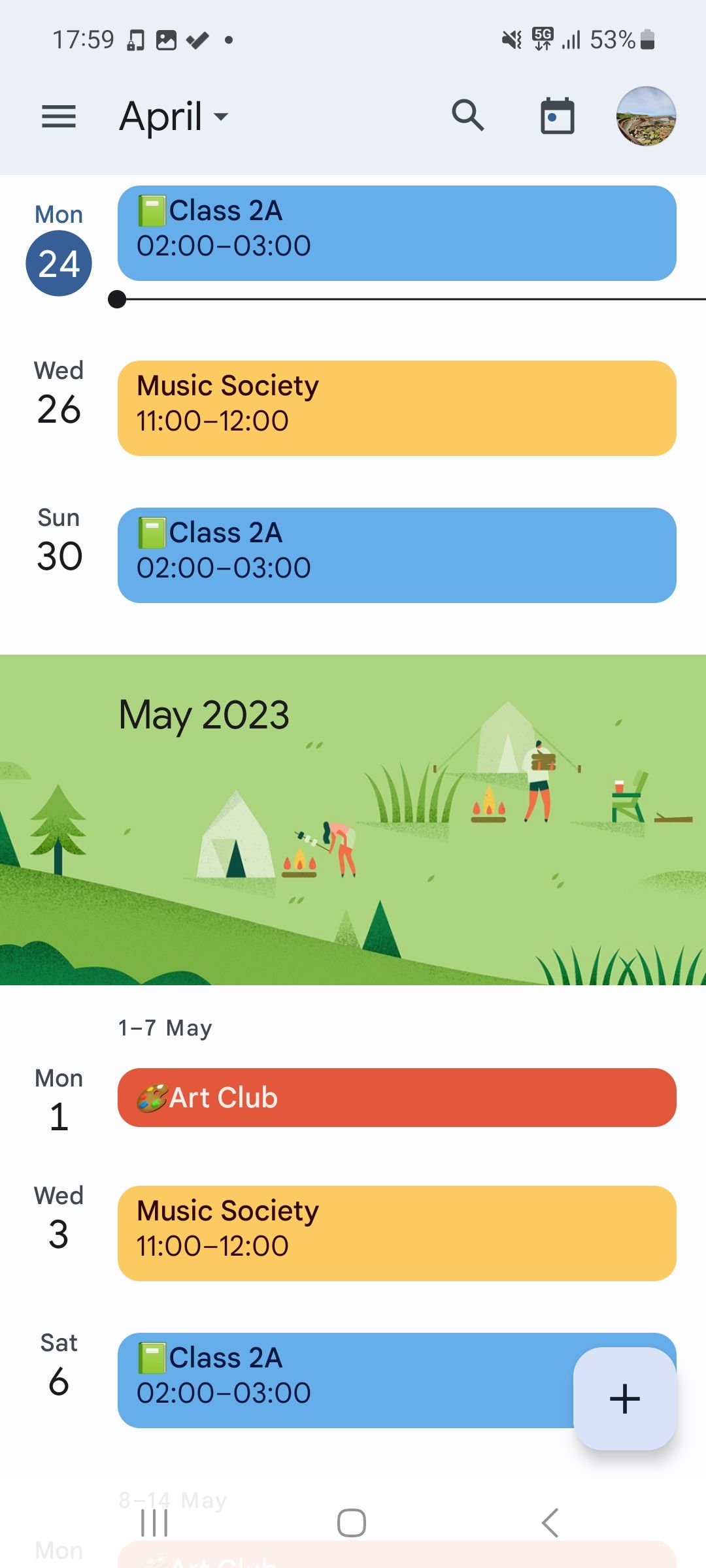A detailed screenshot of a calendar application on a smartphone, set for the month of April. The time displayed at the top of the screen is 17:59. In the upper left-hand corner, identifiable icons include a music note, a screenshot indicator, and a checkmark. On the upper right, there are symbols for vibrate mode, 5G network connectivity, cell phone reception strength, and a battery level at 53%. 

Directly below the icons, a dropdown menu labeled "April" is visible. Listed below are the dates and corresponding events. The dates are arranged vertically on the left side of the screen, beginning with Monday, April 24th, which is highlighted with a blue circle. Events for April include "Class 2A" from 2:00 PM to 3:00 PM on the 24th, "Music Society" on Wednesday, April 26th, and again, "Class 2A" on Sunday, April 30th.

The calendar transitions into May 2023, showing upcoming events: "Our Club" on Monday, May 1st, "Music Society" on Wednesday, May 3rd, and "Class 2A" on Saturday, May 6th.